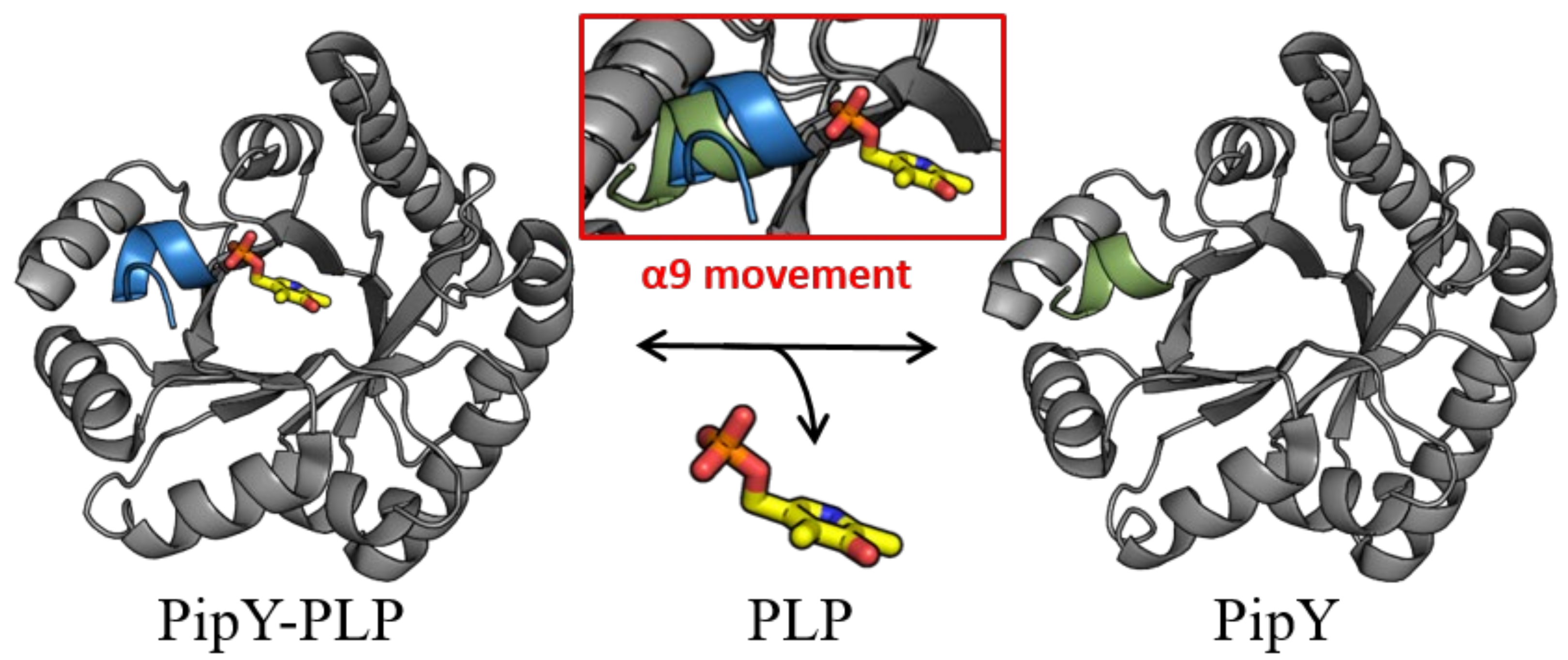This image is a digital illustration, resembling a cartoonish but detailed depiction of a protein obtained from X-ray crystallography. It focuses on the tertiary structure of the protein labeled PIPY-PLP, which features prominent beta sheets and alpha helices, resembling gray metallic coils with sections of blue, red, yellow, and green. The small molecule PLP, characterized by its red and yellow colors and a distinct benzene ring with some substitutions, is embedded within the protein. The inset, labeled "A9 movement," highlights a structural change in the protein as it interacts with the PLP molecule, showing the protein wrapping around the PLP. On the right side of the image, the protein without the PLP molecule, simply labeled PIPY, maintains its coiled structure with green details but lacks the embedded molecule.